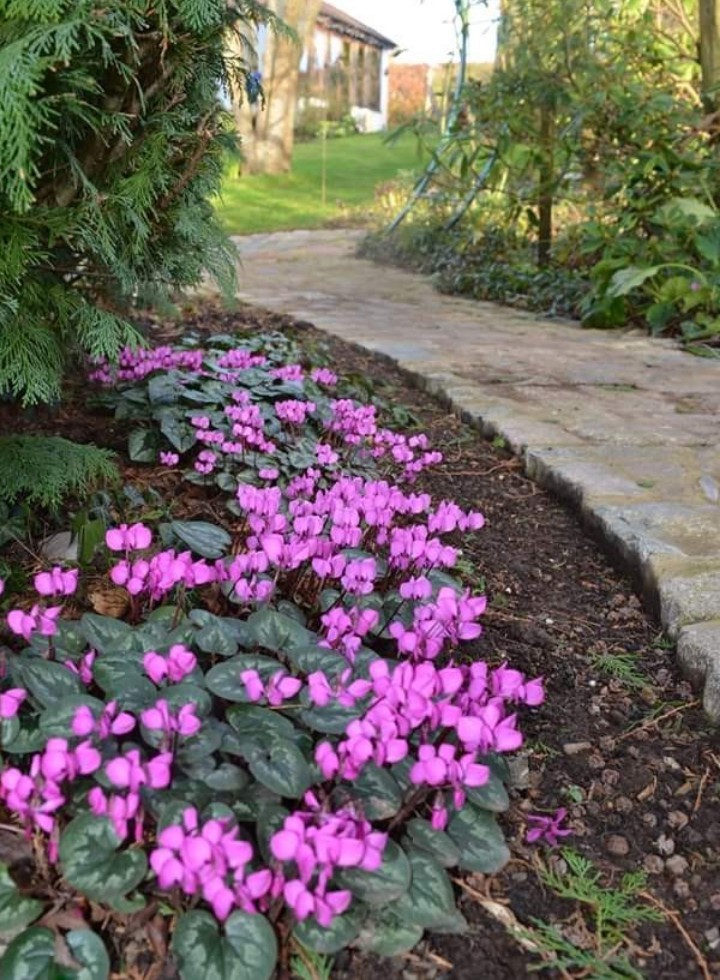The photograph depicts a serene outdoor setting bathed in daylight. Dominating the scene, a stone path meanders through a landscaped area, starting from the center-right and curving gently to the center-left. The pathway is flanked by a well-tended area featuring visible dirt and rocks, indicating meticulous landscaping efforts. On the left side of the image, vibrant flowers in shades of bright pink, fuchsia, and purplish hues punctuate the greenery, their dark, rich colors standing out vividly. Above these blossoms, an evergreen tree adds a lush dimension to the scene.

In the upper-right corner, a tree trunk is visible, surrounded by additional green foliage that enhances the natural feel of the photo. In the far background, partly obscured by vegetation, a house with large windows and a slanted dark roof peeks into view. The bright, sunlit sky overhead appears almost white due to the intensity of the light, emphasizing that the photograph is taken during the day, likely in late spring or early summer when the vegetation is lush and vibrant. The overall focus of the picture appears to be the harmony between the stone pathway, the vivid flowers, and the healthy, green vegetation.